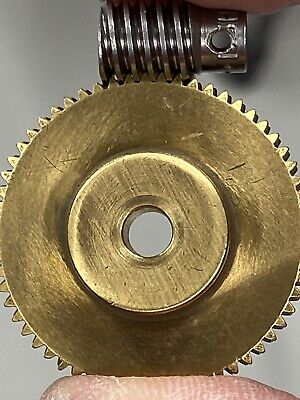The image captures a close-up of a gold, saw blade-like metal object with teeth around its circular edge, held aloft by a person's hand. The outer part of the object is light gold, while the inner part is a darker gold, and it features a central hole, framing the white background behind it. The object, resembling a larger washer or cog used in machinery, is being held between a thumb and another finger. Above the gold piece, there is a silver or gray attachment, likely a screw or sharpener, indicating a sharpening process. The surface of the gold component shines under the light, emphasizing its metallic sheen. The entire setup focuses on the interplay between the golden toothed wheel and its darker attachment against a stark background.